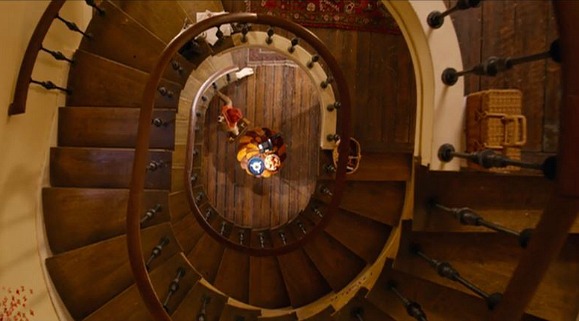This image captures an aerial, top-down view of a beautifully intricate spiral staircase made of dark wood. The staircase spirals down at least three times, encased by a matching dark wood railing interspersed with vertical iron slats for added support and aesthetic appeal. At the bottom of the staircase, the wooden floor is visible, partially illuminated by a source of light placed on an orange object—which is ambiguous but could convincingly be a table. To the right of this object, there is a hint of something that appears to be a bowl, though it's distant and not entirely clear. On the top left, there's a glimpse of a person with red hair, likely a woman. Towards the far right, at one loop of the stairs, a tan wicker bag with handles is casually set down. The scene combines the elegance of the staircase's design with subtle, intriguing details at its base.